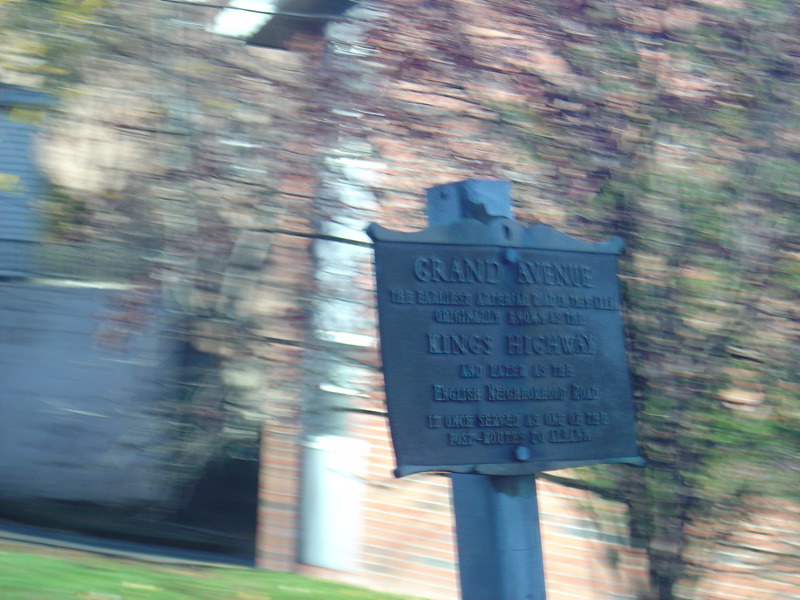This is a very blurry outdoor photograph taken in the afternoon, possibly from the vantage point of a passing car or a pedestrian near the curb. In the foreground, there is an ornate, antique-looking cast iron sign mounted atop a metal rectangular post. The sign, which appears dark black or dark gray, features embossed letters. It prominently displays "Grand Avenue" at the top, followed by smaller, partially legible text that includes "Kings Highway" and possibly "English Neighborhood Road." The sign seems to be indicating a historical marker, with further writing that is difficult to decipher due to the image's blur.

In the background, there is a brick building with a light red hue, partially covered by a black mesh fence. Some ivy might be growing up its side. There is green grass visible in the lower left corner of the image, along with a tall tree that is beginning to shed its leaves, suggesting it could be fall. The overall scene is impromptu and blurry, lending a sense of motion or momentary capture to the photograph.